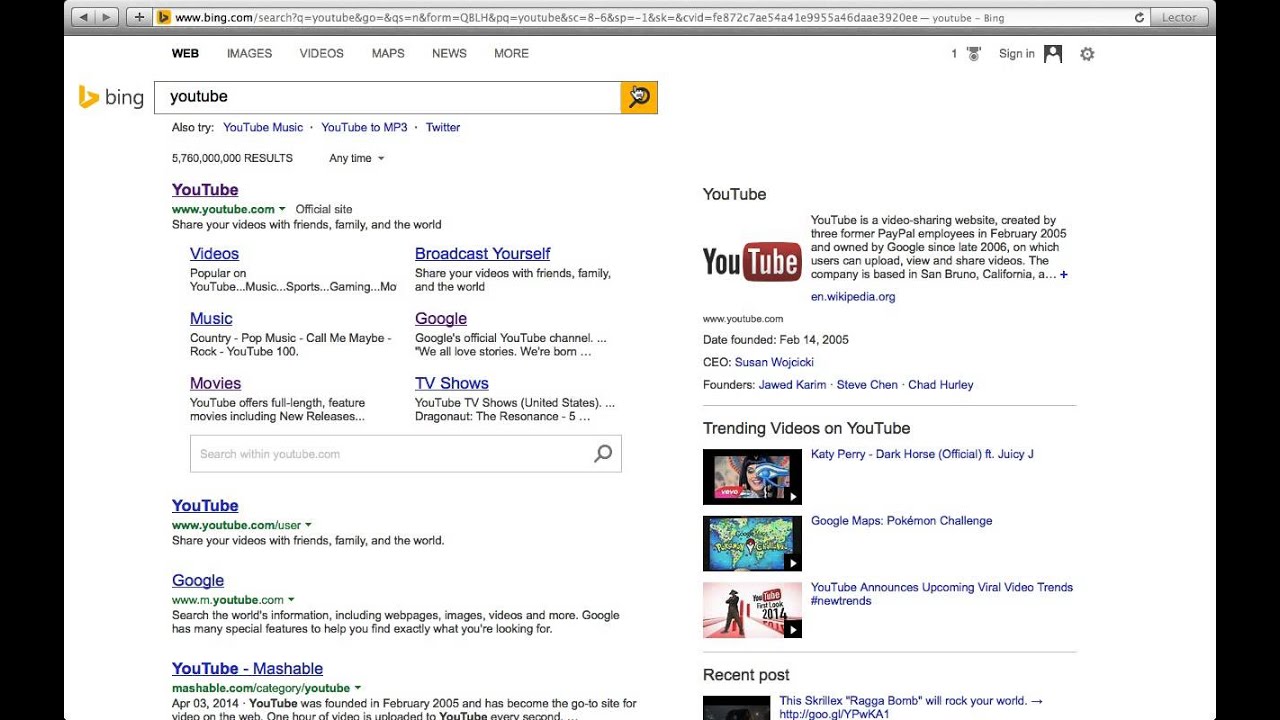The image depicts a computer screen displaying the Bing search engine homepage. At the very top, there is a typical web browser address bar showing "www.bing.com" along with a string of additional search parameters. Below the address bar, the main Bing interface is visible. 

The page is primarily white in color and organized with navigational options at the top. These options include "Web," "Images," "Videos," "Maps," "News," and "More," with "Web" currently highlighted in bold. The Bing logo is prominently displayed next to the word "Bing."

There is a central search bar on the screen, with the word "YouTube" already typed into it. A yellow search button featuring a magnifying glass icon is situated next to the search bar, with the mouse cursor hovering over this button.

Underneath the search bar, Bing suggests related topics including "YouTube Music," "YouTube to MP3," and "Twitter." The search query has yielded approximately 5,760,000,000 results. 

The first search result listed is the official YouTube website, described as a platform to "share your videos with friends, family, and the world." Beneath this description, there are hyperlinks to specific YouTube categories such as "Videos," "Music," "Movies," "Broadcast Yourself," "Google," and "TV Shows." Additionally, there is another search bar within this result to conduct searches specifically on YouTube.com.

Further down the page, there are more clickable search results including "YouTube" and "Google" and another link to "YouTube Mashable." On the right-hand side of the screen, at the top, an option to "Sign In" is visible. Further information about YouTube is provided, including the platform's founding date, February 14, 2005. Below this, there are sections highlighting trending videos on YouTube.